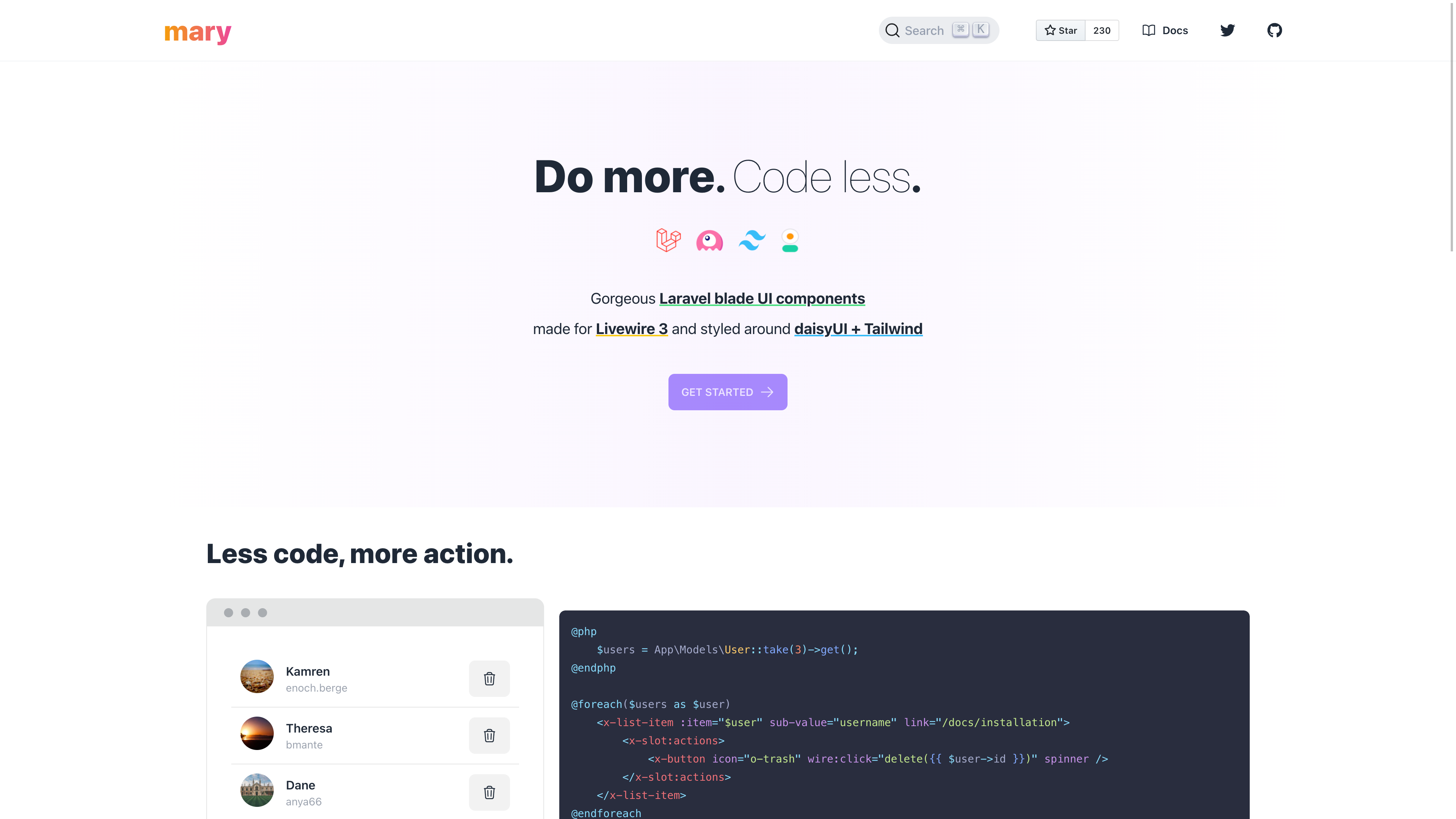The image depicts a computer webpage designed for a user named Mary, whose name appears in the upper left-hand corner in a text that transitions from orange to pink. At the top, there's a search bar for easy navigation. Below this, a prominent message reads "Do More, Code Less." Beneath this slogan are several icons accompanied by text that appears to say "gorgeous, leveled blonde little components, made for You Wake 3 and styled around Daisy UL." 

Additionally, there’s a mention of "talk wind" or possibly "tall wind," written nearby. A purple box is displayed underneath these elements. Further down the page, a section reads "Less Code, More Action," and features profile images of three individuals identified as Theresa (center), Kareem, and Donny (or possibly Dom). 

Next to these profiles is a black box containing multicolored text in red, yellow, green, and purple, which is difficult to read due to the dark background. The webpage has a small print and appears to be tailored specifically for Mary.